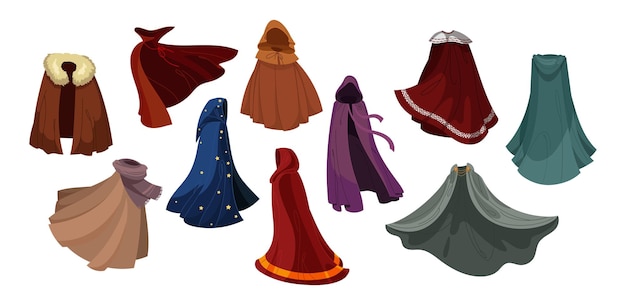The image features a horizontally rectangular composition comprised of a collection of ten illustrated capes, cowls, and robes set against a clean white background, emphasizing their design without distraction. Displaying an array of vibrant colors, textures, and styles, these artistic drawings depict garments that could be layered over regular clothing.

Starting from the left, there are two brown cloaks: one adorned with a fur-lined collar and the other with a scarf wrapped around it. Positioned slightly in front of these, there's a deep blue robe with star motifs, reminiscent of a wizard’s attire. Moving towards the center, a grey cloak and a red cloak—both plain in design—are set side by side. Above these, there is another brown garment.

Further to the right, a rich purple robe and a crimson cloak with white trim along the bottom stand out. A distinctive green cowl with a chain closure around the neck is placed next, followed by a teal piece of cloth on the far right, which wraps around the neck with an attached scarf for securing. The artistic drawing showcases a blend of fabrics including fur, leather, and brocade, alongside varying decorative elements like stars, hoods, and collars, capturing the versatility and imaginative craftsmanship of these conceptual designs.